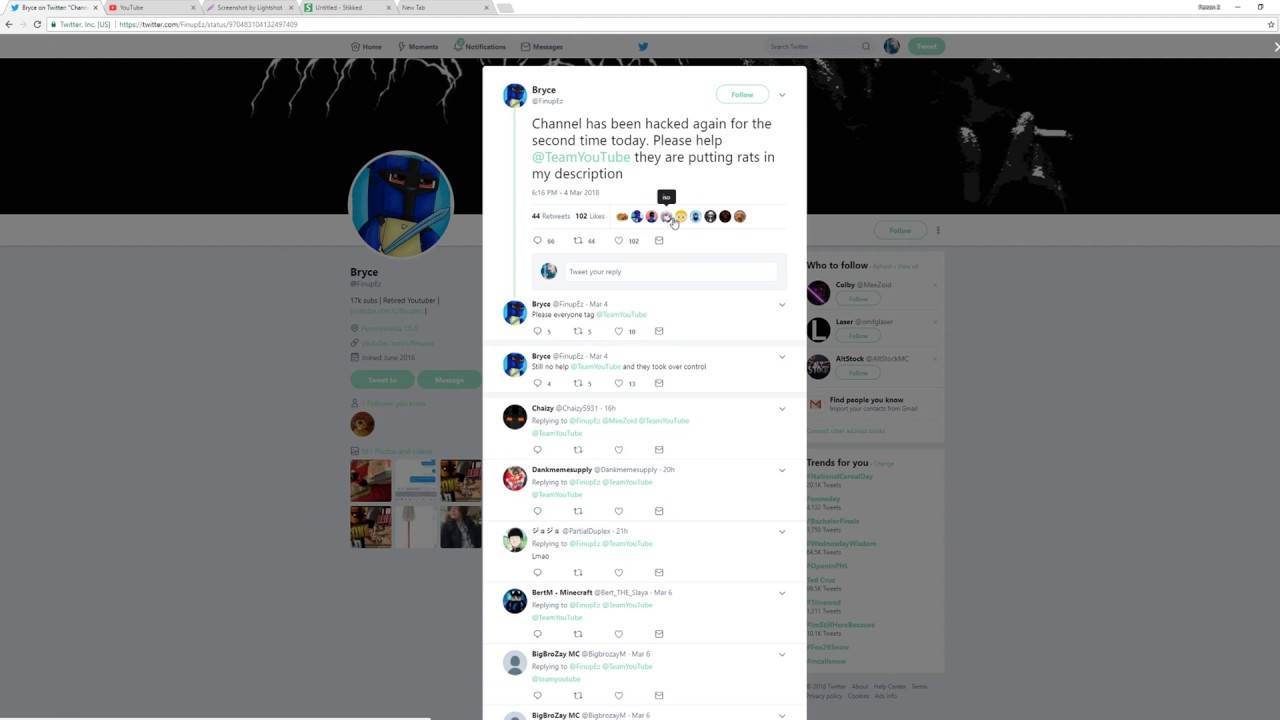The image showcases the Google Chrome browser with multiple tabs open. The primary tab displayed is the Twitter app. Along the top, various tabs are visible, including Twitter, YouTube, Lightshot for screenshots, an untitled document, and a new tab.

The main Twitter tab features the profile of a user named Bryce. Visible elements of Bryce's profile include parts of their profile picture and banner image, along with some basic information that states "17k subs, retired YouTuber." Links to their YouTube channel and their location details are also partially visible, along with a few of their tweets, which are not fully clear.

Dominating the foreground is a specific tweet from Bryce. The tweet reads: "Channel has been hacked again for the second time today please help @TeamYouTube they are putting rats in my description." Beneath this tweet, there is a series of replies, including another tweet from Bryce urging followers to tag @TeamYouTube, along with responses from other users tagging @TeamYouTube and additional contacts in an effort to draw attention to the issue.